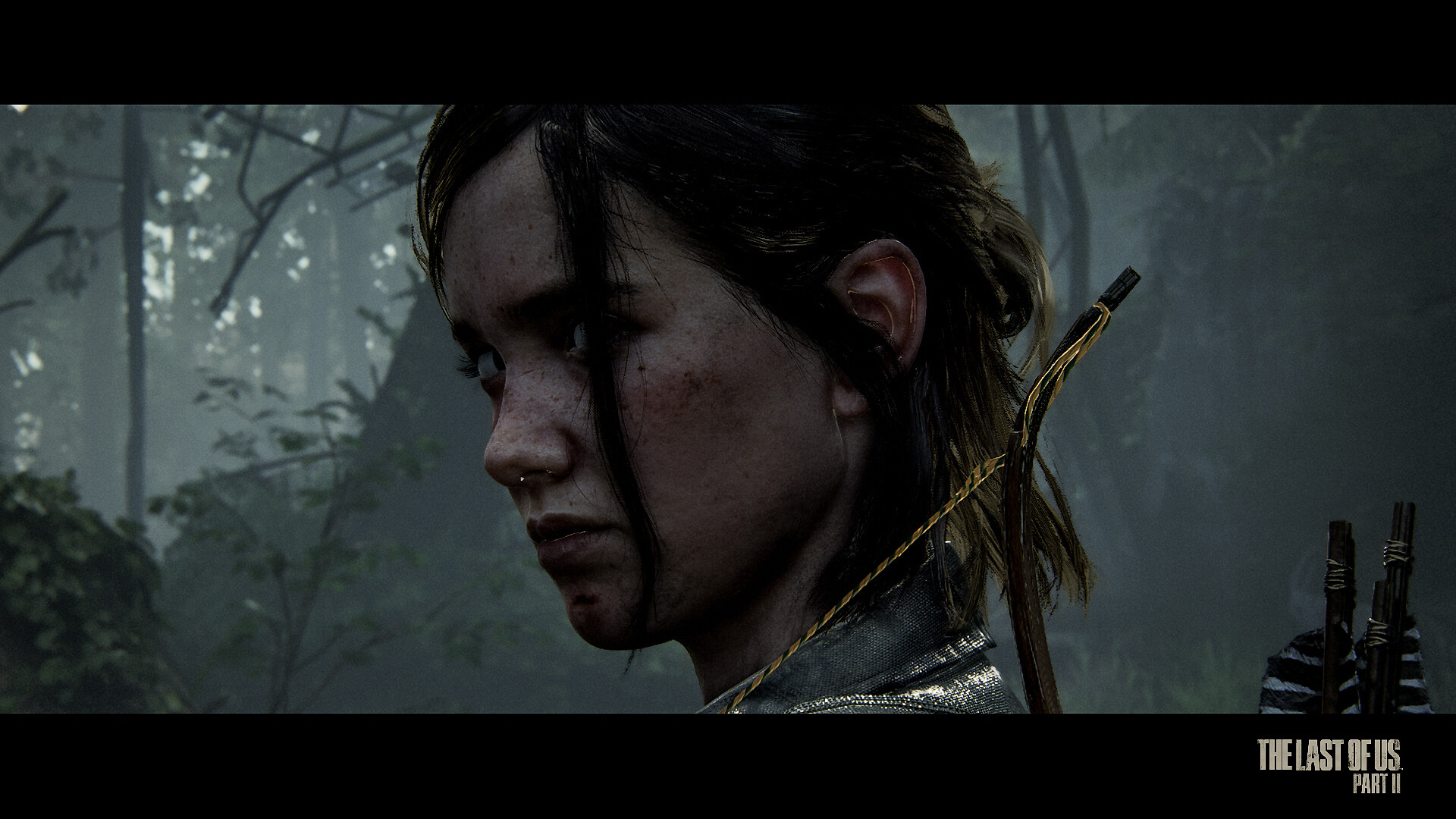This is a promotional image for the video game The Last of Us Part 2. The horizontal image features black bars on both the top and bottom. In the lower right corner, within the black border, the title "The Last of Us" is prominently displayed in large white letters, with "Part 2" in smaller text below it. The background is dominated by a dense forest scene, with numerous trees, branches, and leaves. A bit of light filters through the foliage on the left side, adding a touch of brightness to the otherwise muted scenery.

Centered in the image is the head and upper shoulders of a young girl, who appears to be looking over her left shoulder with a mix of fear and anger. Her dark hair is worn up but falls in strands that partially cover her left eye. Her face, which carries a few nicks and abrasions, is dirty and worn, suggesting she's been through tough situations. A distinctive strand of gray hair drapes across her face. She has a nose piercing and is wearing a shirt with a visible silver collar, though the rest of the shirt is cut off from view.

The girl is carrying a bow over her left shoulder, with a yellow and black string visible just below her ear. A brown stick, part of the bow, curves up from the bottom and is adorned with a gold feather at the top. In the right corner of the image, three wooden arrows with black and white fletchings emerge, indicating that they are housed in a quiver over her shoulder. The atmosphere is enhanced by a subtle mist and white skies in the distance, adding to the overall tension and mood of the scene.